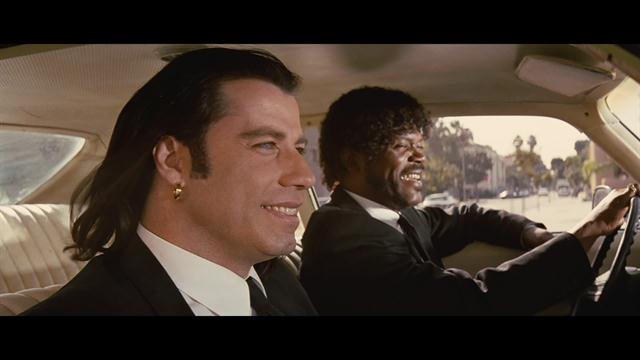This image is a still shot from the iconic movie "Pulp Fiction," featuring Samuel L. Jackson as Jules and John Travolta as Vincent. They are seated inside a vintage car with a cream leather interior that evokes a 70s feel. Samuel L. Jackson, with his distinctive afro and curly hair, is at the wheel, his hand resting casually on the window sill. Both characters are dressed sharply in suits; Jules in a classic ensemble and Vincent distinguished by his long, dark, flowy hair and a noticeable gold earring. The background through the windshield reveals a typical Los Angeles street scene, with buildings, cars, and greenish-yellow trees under an overcast sky. The shot captures them mid-conversation, both smiling and seemingly happy, as Vincent animatedly explains the cultural idiosyncrasies of Amsterdam and Europe, famously referring to the "Royale with Cheese" and other food-related differences.